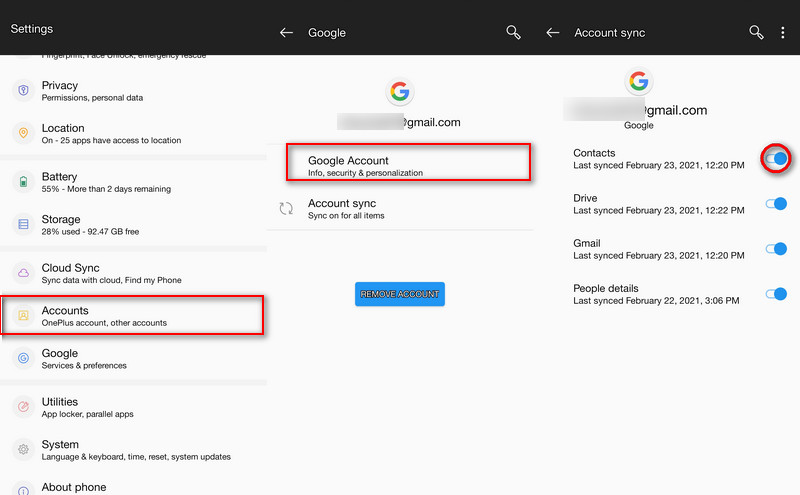The image depicts a settings page of an individual's Google account. At the top of the page, a black bar features various navigation elements. On the upper left-hand corner in white text, the word “Settings” is displayed, followed by a left-facing arrow and the word “Google.” To the right of this, there is a search icon, another left-facing arrow, and more text reading “Account Sync.” Additionally, there is another search icon and a vertical ellipsis (three dots) icon.

Beneath this header, the background transitions to white, organizing the content into three distinct columns. 

- **Center Column:** Dominating this section is the Google logo, represented by a white circle with a multi-colored 'G' in the center. Beneath the logo, only the domain “gmail.com” is visible, as the person's name is deliberately blurred out for privacy reasons. Directly beneath this, there are various navigation links, including “Google Account,” “Info,” “Security,” and “Personalization,” encapsulated within a red rectangle, drawing attention to this area.

- **Right Column:** Similar to the center column, this area features another circle with the multi-colored 'G.' Adjacent to it, the individual’s name appears blurred next to “gmail.com.” Below, there is a section labeled “Contacts” highlighted by a toggle switch, which is currently in the 'on' position and encircled by a red rectangle, indicating its active status.

The caption comprehensively details the structure and elements of the Google account settings page, offering a clear visual description for those unable to see the image.